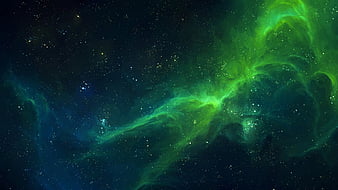This image depicts the Aurora Borealis, also known as the Northern Lights, set against a dark, midnight blue sky. It is a small, low-resolution, rectangular photo, capturing a striking natural phenomenon. The sky is filled with numerous faint, star-like specks that add a touch of celestial beauty. Dominating the scene is a vibrant, green to bluish gradient haze that stretches from the lower left to the upper right corner, resembling a spray-painted effect. This luminous display forms a series of lines with hazy edges that contrast starkly with the deep blue night sky, making it an exceptionally beautiful and visually captivating subject. The green glow, typical of the aurora, vividly stands out and adds an element of ethereal charm to the overall composition.